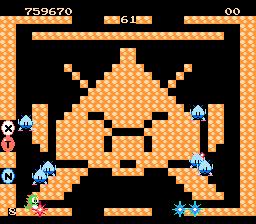The image depicts an old-school video game, likely Bubble Bobble, characterized by pixelated 8-bit or 16-bit graphics. Dominating the image is a black background bordered with orange blocks. These blocks create an almost complete border with gaps leading to a possible kill screen. Centrally, the blocks form a large, turnip-like alien figure with a triangular head, 45-degree angle antennae, blocky arms, and legs, as well as a simple face featuring eyes, a nose, black eyebrows, and a small mouth.

Surrounding this central figure are six smaller, similar creatures. These smaller characters are half blue on the top and dark blue on the bottom, spread out three on each side of the central figure. Additionally, a small green dinosaur-like character, reminiscent of a tiny Godzilla with a white belly and orange spikes, is positioned lower in the image.

On the left-hand border sit three colored circular objects: a white circle with a black X, a red circle with a black T, and a blue circle with a black N. The game's interface displays a score of 759,670 in the upper left, a timer reading 61 in the middle, and a second score of zero in the upper right, suggesting it could be for a second player. Sparkly objects that might be jewels or stars float within the game’s environment, adding to its retro charm.